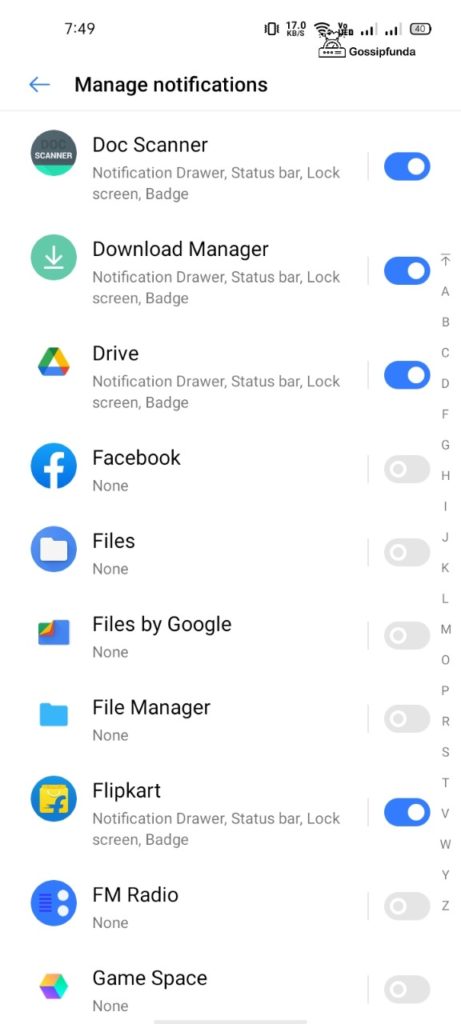This screenshot depicts a mobile application interface specifically designed for managing notifications for individual apps. In the upper left-hand corner, the time is displayed as 7:49. Stretching from the center to the right-hand side of the status bar, there are several icons, including the Wi-Fi signal strength indicator, cellular signal strength indicator, and a battery icon displaying 40% charge.

The screen's heading, "Manage Notifications," is prominently featured at the top, accompanied by a blue left arrow situated to the left of the bold black text. Below the heading, a list of various apps is presented, each with options to toggle notifications on or off. The active toggles are indicated in blue, while inactive toggles are gray.

To the right of the app list, an alphabetical index (A to Z) is vertically aligned, serving as a shortcut for quick navigation through the list of apps. The displayed apps and their respective notification statuses are as follows:

- Dock Scanner: Notifications toggled on (blue)
- Download Manager: Notifications toggled on (blue)
- Google Drive: Notifications toggled on (blue)
- Facebook: Notifications toggled off (gray)
- Files: Notifications toggled off (gray)
- Files by Google: Notifications toggled off (gray)
- File Manager: Notifications toggled off (gray)
- Flipkart: Notifications toggled on (blue)
- FM Radio: Notifications toggled off (gray)
- Game Space: Notifications toggled off (gray)